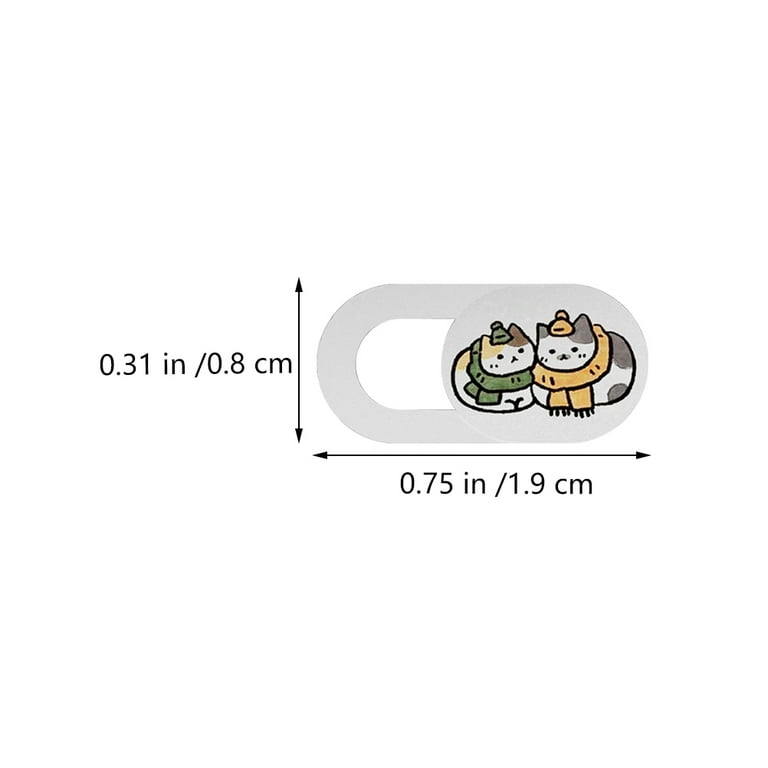The image is an animated depiction featuring two cats. The larger cat, positioned on the right, has gray and white fur, and wears a yellow hat and a matching yellow scarf. The smaller cat, standing next to it, has a coat of yellow, white, and brown fur, and is adorned with a green hat and green scarf. The background sets a mechanical tone, resembling the face of a combination lock outlined in gray with a central white space. To the left and underneath, there are measurement indicators, with an arrow pointing to the left measuring distances. On the left side, it reads "0.31in / 0.8cm," and below that, it reads "0.75in / 1.9cm." The overall composition combines a playful depiction of the cats with a precise, almost technical backdrop.